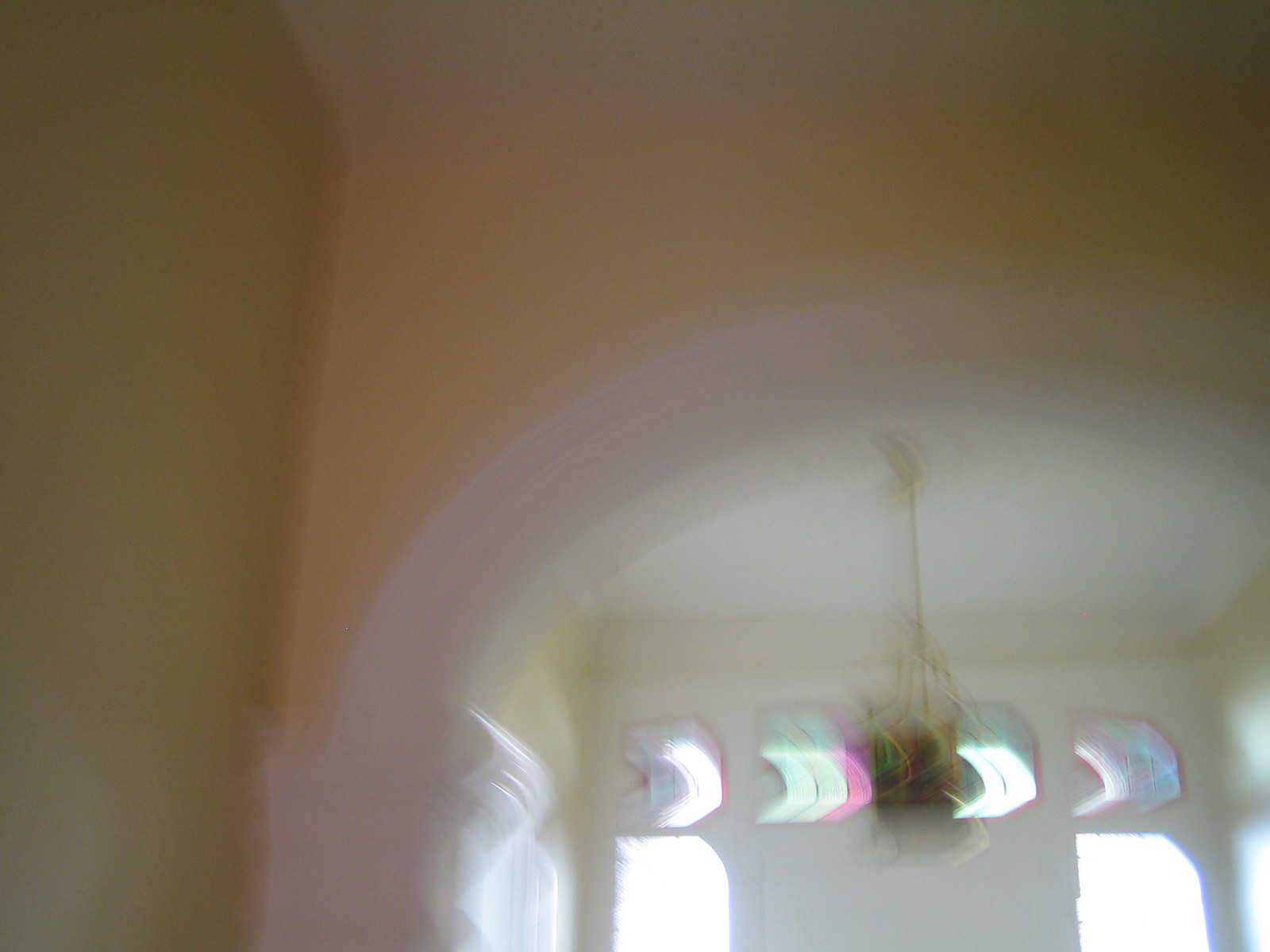This image depicts the interior of a house, captured from a height of approximately six to seven feet. The focus of the image is an arched doorway leading into another room within the house. The photograph is noticeably blurry, suggesting it was taken either while the camera was in motion or not properly focused. In the background, there are several windows allowing natural sunlight to stream into the space. Overall, the scene is characterized by its indistinct quality and the sense of an accidentally taken picture.